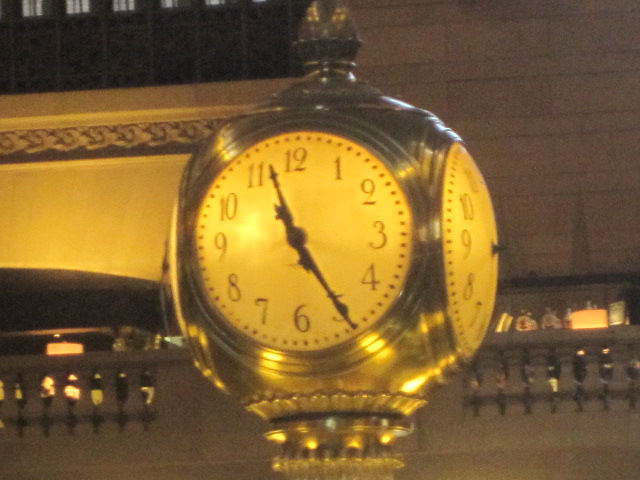The image showcases a street-side clock with four faces, oriented towards the left, right, front, and back, ensuring it's visible from any direction. The clock’s faces have a gold hue, adding a timeless elegance to its appearance. The clock is mounted on a column, though the base of the column is cut off in the frame. In the background, a building dominates the scene, accompanied by a parked car partially visible on the left-hand side. The entire image is bathed in a warm, golden filter, enhancing the vintage and atmospheric quality of the scene.